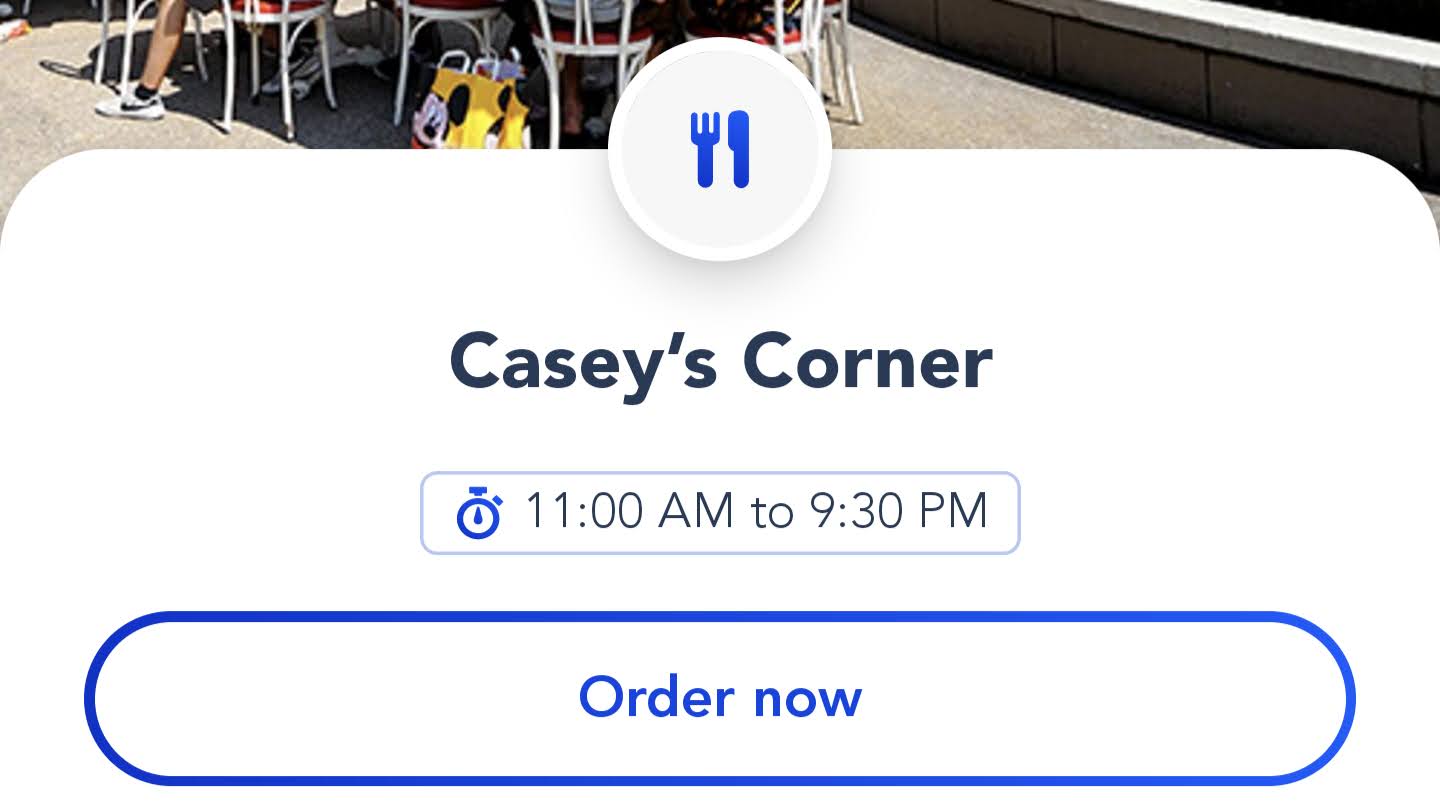The image captures an outdoor scene at Casey's Corner, prominently featuring a page design that highlights key information about the restaurant. At the top of the page, within a white circle, there is an icon of a blue fork and knife. Beneath this icon, "Casey's Corner" is written in bold black text. Below, a blue-bordered square displays the restaurant's operating hours, "11am to 9:30pm," and an inviting "Order Now" button in blue.

The background reveals the exterior dining area on a sunny day. Visible reflections suggest bright sunlight, and a gray wall forms the backdrop. The floor is concrete, and the seating consists of white chairs with red cushions. Several guests are shown enjoying their meals, with one noticeable detail being a yellow Mickey Mouse bag with white handles lying on the ground. A person can be seen wearing black socks paired with white and black sneakers, while other diners have placed their belongings, such as bags, under the tables. The atmosphere is lively, characteristic of a bustling restaurant offering food to its patrons.